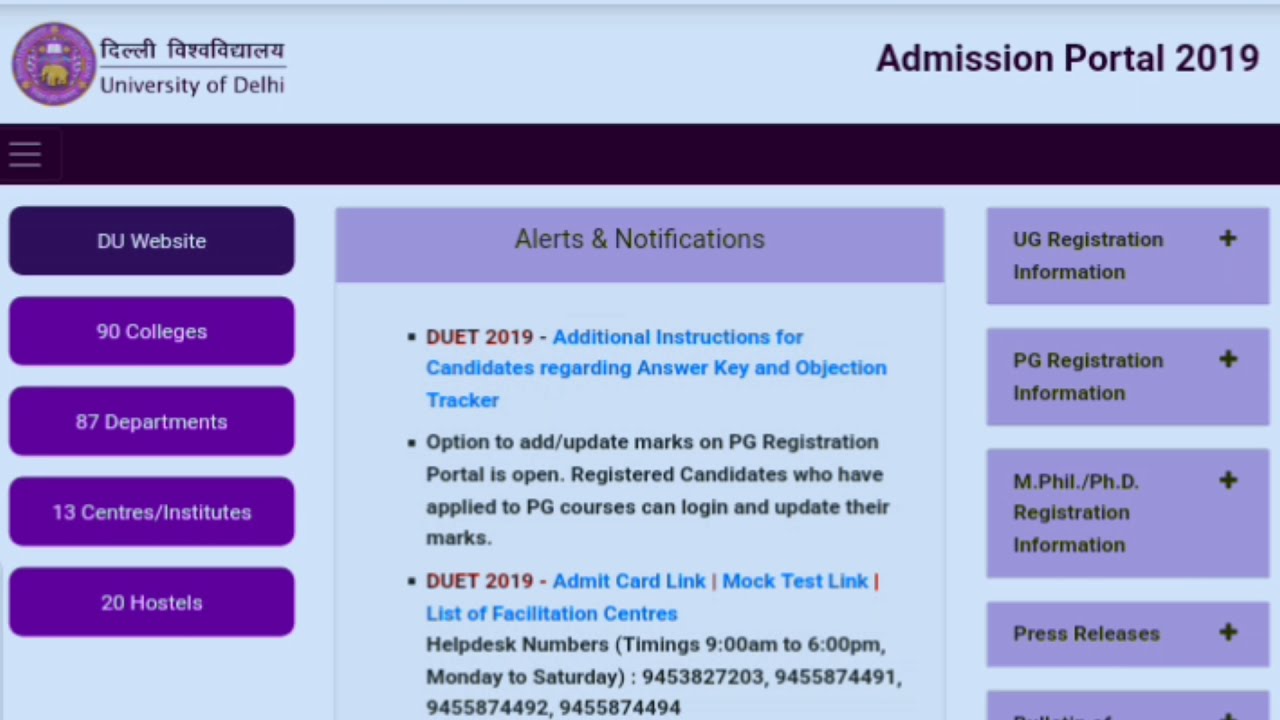This screenshot captures the University of Delhi's Admission Portal 2019, characterized by a vibrant color scheme including purple, pink, light blue, white, black, and red. Positioned in the top left is the university's logo, a purple circle featuring a yellow elephant emblem likely representing the college's coat of arms. Adjacent to the logo, the text "University of Delhi" is prominently displayed in purple on a light blue background.

Beneath this heading, in larger black font, "Admission Portal 2019" stands out at the top center of the webpage. The left side of the screenshot features vertical navigation links including "DU website," "90 colleges," "87 departments," "13 centers/institutes," and "20 hostels."

Central to the image is a dark band displaying a three-line menu icon, below which, in a purple background with black text, the headings "Alerts and Notifications" and "Duet 2019" appear. Additional text in various colors reads, "Additional Instructions for Candidates Regarding Answer Key and Objection Tracker," followed by "Option to Add or Update Marks on PG Registration Portal is open. Registered candidates who have applied to PG courses can log in and update their marks." 

Further down, the words "Duet 2019" appear again in red, accompanied by "Admit Card Link," "Mock Test Link," and "List of Facilitation Centers" in blue. The right-hand side of the screenshot is divided into sections with labels like "UG Registration Information," "PG Registration Information," "MPhil/PhD Registration Information," and "Press Releases," each marked with a plus sign. Everything is well-spaced, resulting in a clear and organized layout, typical of a university website.